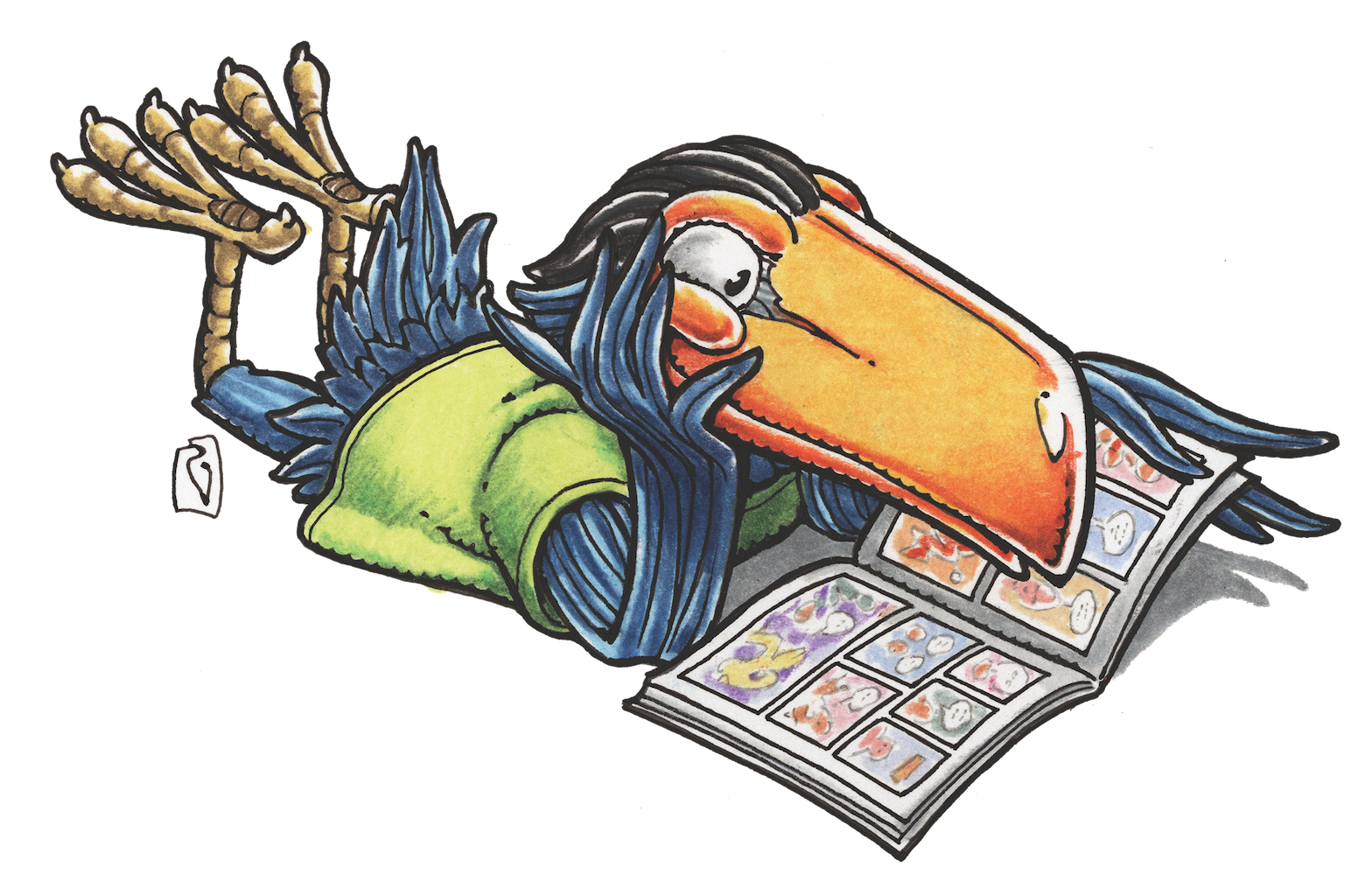The illustration depicts a cartoon toucan leisurely reading a comic book. The toucan is laying on its stomach with its legs kicked up in the air, mimicking a relaxed, human-like pose. It is deeply immersed in the book, holding its head with one hand (or wing) while the other wing holds the book open. The bird is adorned with dark blue feathers, a bright neon green t-shirt, and tan or brown legs and feet. Its most striking feature is a large, bright orange beak that is almost half the size of its body. The toucan's eyes are focused and intent, giving the impression of curiosity or enjoyment. The comic book features multiple illustrations but no visible text, suggesting a visually driven narrative. The background is plain white, emphasizing the character and its actions. Additional details include black, slicked-back feathers on its head and an artist's signature, indicating it is a unique, hand-drawn piece, possibly created with markers or colored pencils.